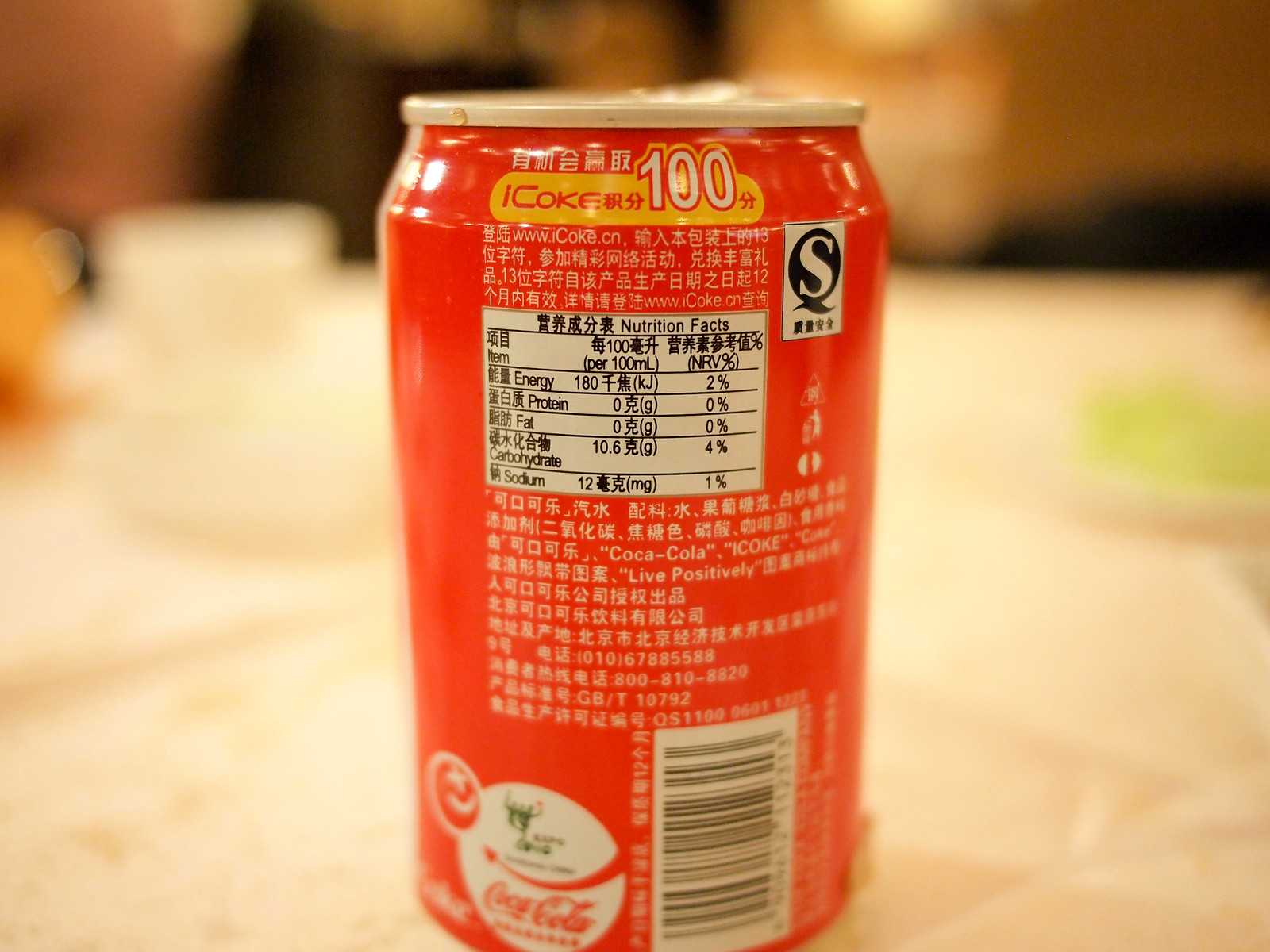This is a close-up photograph of a red Coca-Cola can featuring Japanese writing. The can has a silver top and bottom rim, with a prominently visible white circle on the front, through which a red arrow points to the left. Also noticeable on the front is a red circle with a white border and an 'X' symbol featuring a crescent moon-like shape. The branding includes the word "Coca-Cola" in red text within the large white circle, and an English website, www.coke.cn. The can displays a UPC barcode in a white rectangle with black stripes. The label includes detailed nutrition information in black font on a white background. The background of the image is blurred, with the can standing upright on a white countertop, and some indistinct, blurred objects appearing on the left side.